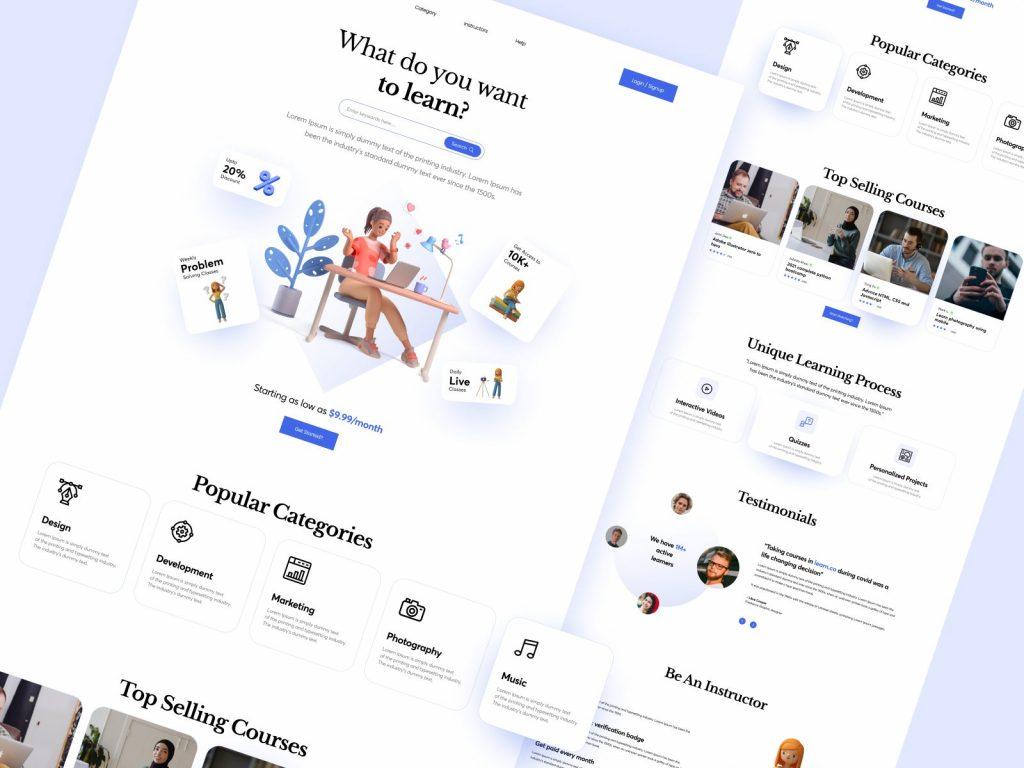The photograph depicts an assortment of brochures or website mockups related to an online learning platform, laid out in a slightly tilted, right-slanted arrangement. Poised at the top of one of the prominent pages is the question, "What do you want to learn?" accompanied by a search bar for user queries. The page also features placeholder text, reading "Lorraine is simply dummy text of the printing industry," suggesting customizable content areas. 

In addition, the layout showcases a myriad of emojis and snippets, including enticing offers like "Get access to 10K+ courses," "20% deliverable," and "Weekly problem-solving classes." Under the "Popular Categories" section, disciplines such as Design, Development, Marketing, Photography, and Music are spotlighted. The page also highlights "Top Selling Courses," details about the "Unique Learning Process," and testimonials. Educational methodologies are elaborated upon under the "Unique Learning Process," which mentions interactive videos, quizzes, and personalized projects, underscoring the platform's commitment to engaging and individualized learning experiences.